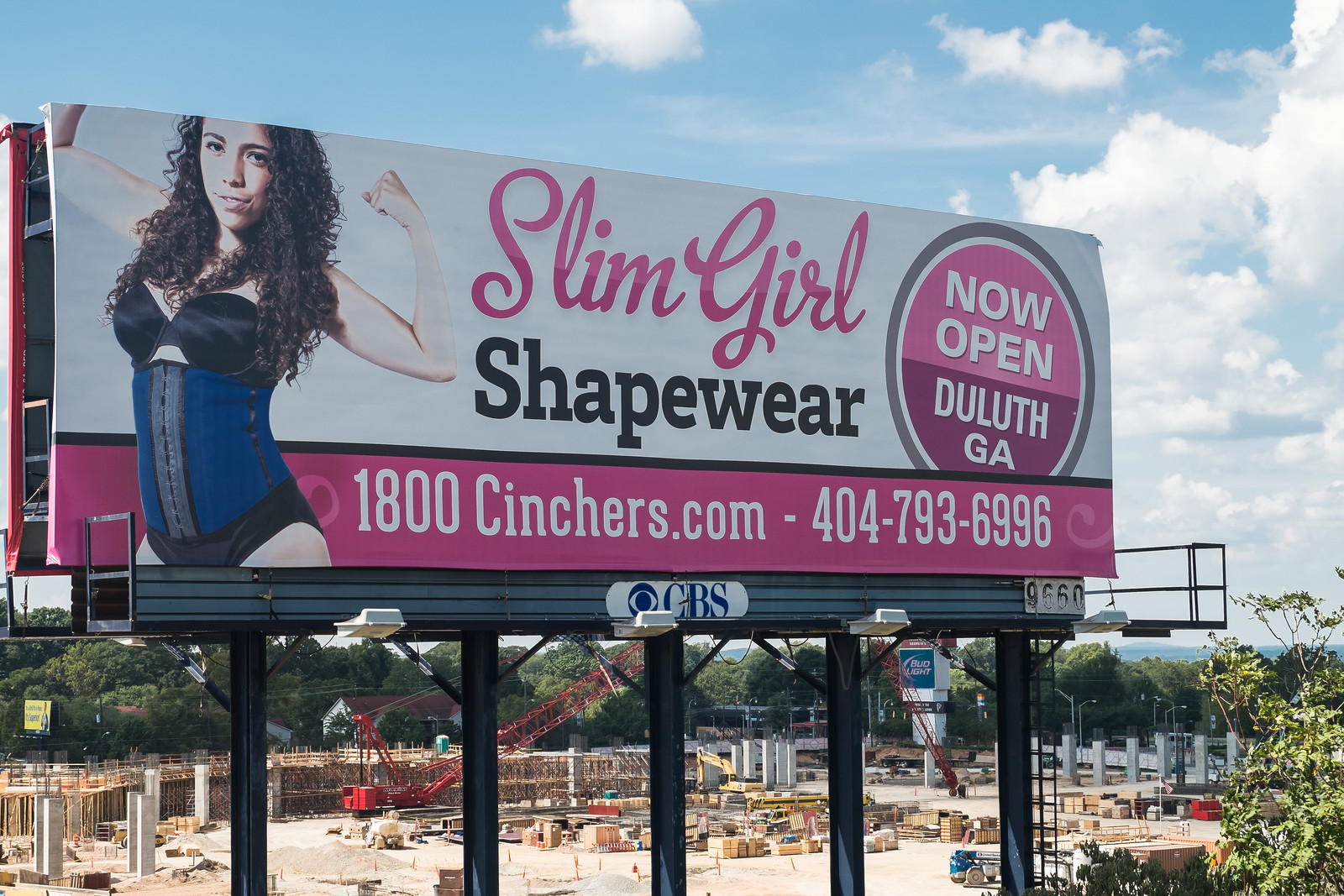This daytime photograph captures a billboard prominently displayed against a backdrop of sky and clouds. Below the billboard, a construction site is visible, featuring various concrete columns and wooden scaffolding. 

The billboard itself has a predominantly white and pink color scheme. It advertises "Slim Girl Shapewear," stating "Now Open, Duluth, GA" in clear serif and sans-serif fonts. The contact information includes a phone number, 404-793-6996, and the website, 1-800-CINCHERS.COM, with "1-800-CINCHERS" set against a pink background.

A central image on the billboard features a Caucasian woman with black curly hair, flexing confidently. She is wearing blue shapewear along with a black bra and panties. The text "Slim Girl" is written in a pink, curly script whereas the rest of the text uses serif and sans-serif fonts, creating a visually distinct and engaging advertisement.